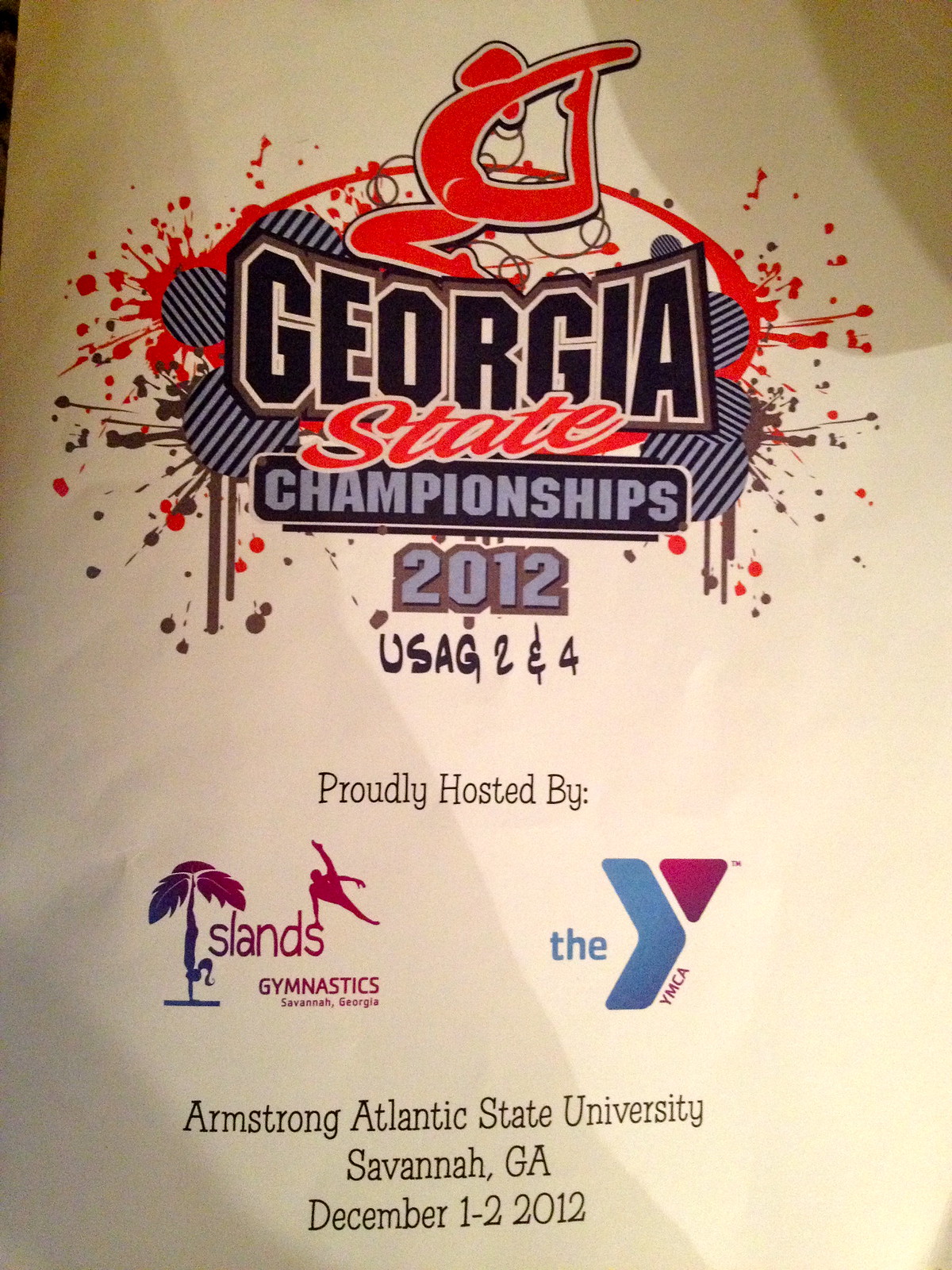This detailed caption describes a promotional poster for the Georgia State Championships 2012 in gymnastics, proudly hosted by Islands Gymnastics of Savannah, Georgia, and the YMCA. The event took place at Armstrong Atlantic State University in Savannah, Georgia, from December 1st to 2nd, 2012. The poster features a striking design with a gymnast figure in orange positioned above the text, encapsulating a gymnastic pose with her right hand touching her upturned left leg. The text "Georgia" appears in black, followed by "State" in red, and "Championships 2012" underneath, collectively reading "Georgia State Championships 2012." The poster has a reddish-brown gradient background on the upper section with artistic splatters accentuating the theme, while a lighter brown section below contains advertisements. The Islands Gymnastics logo, with a palm tree and a gymnast, adds to the event’s branding, and the YMCA logo prominently features its distinctive blue and purple "Y." This vibrant and engaging poster serves as both a promotional tool and memento for the exciting state-level gymnastic championship event.